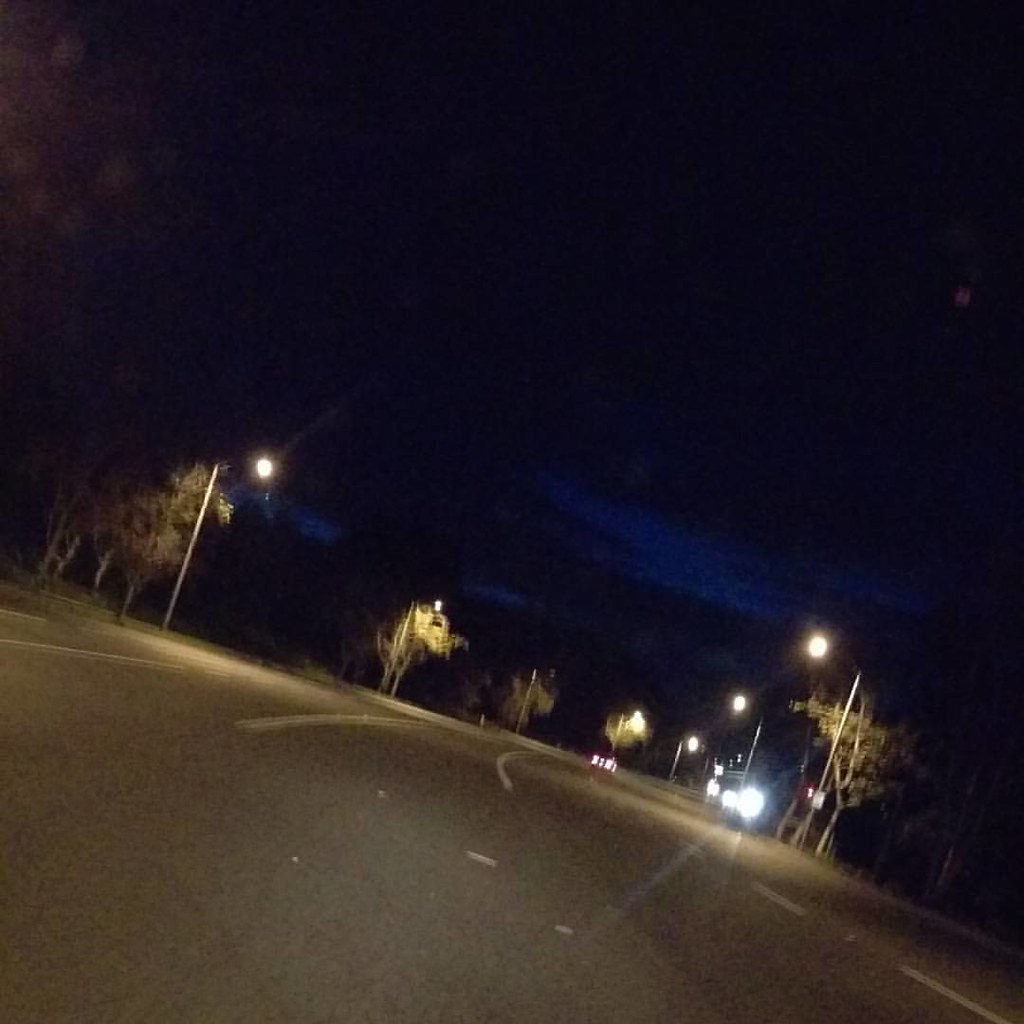A nighttime photograph taken from inside a car captures a wide, almost deserted, three-lane road heading straight before curving slightly to the right. The sky is a dark, cloudy blue, creating pockets of light that contrast with the nearly pitch-black areas. Along both sides of the road, streetlights cast warm glows, highlighting sporadically placed trees standing close to the curb. Street signs and traffic lights are also visible, with one directly overhead of the road. A single car with one headlight brighter than the other is seen far ahead. White lines on the road guide the curve, and distant round lights, possibly from another car, appear slightly to the right, adding depth to the scene.